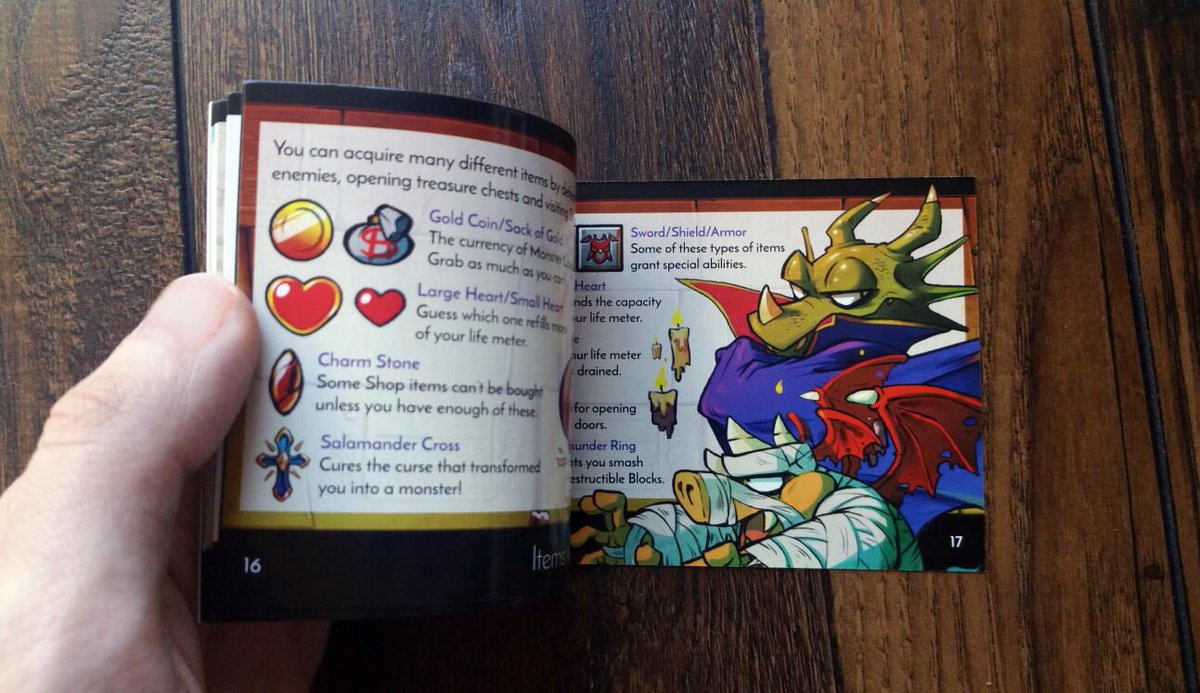This image captures a hand thumbing through a small instruction booklet that resembles one included with old Nintendo video games. The booklet is open to pages 16 and 17, though page 16 is partly obscured. The visible text on page 16 starts with "you can acquire many different items by," but is cut off by the curve of the pages. What can be read mentions items obtainable through defeating enemies, opening treasure chests, and possibly other unreadable actions. Illustrated items include a gold coin, a sack of gold, a large heart, a small heart, a red gem labeled "charmstone," and a cross with two spikes labeled "salamander cross." Positioned on a dark brown wooden surface, the booklet's right page details more items and features cartoonish, high-contrast illustrations. Highlighted are a dark green dragon with a spiked snout, wearing a vampire-like purple and red cape, and a pig-like creature garbed in mummy bandages, with horns and red wings tipped with spikes. The shield pictured on this page is labeled "sword slash shield slash armor."